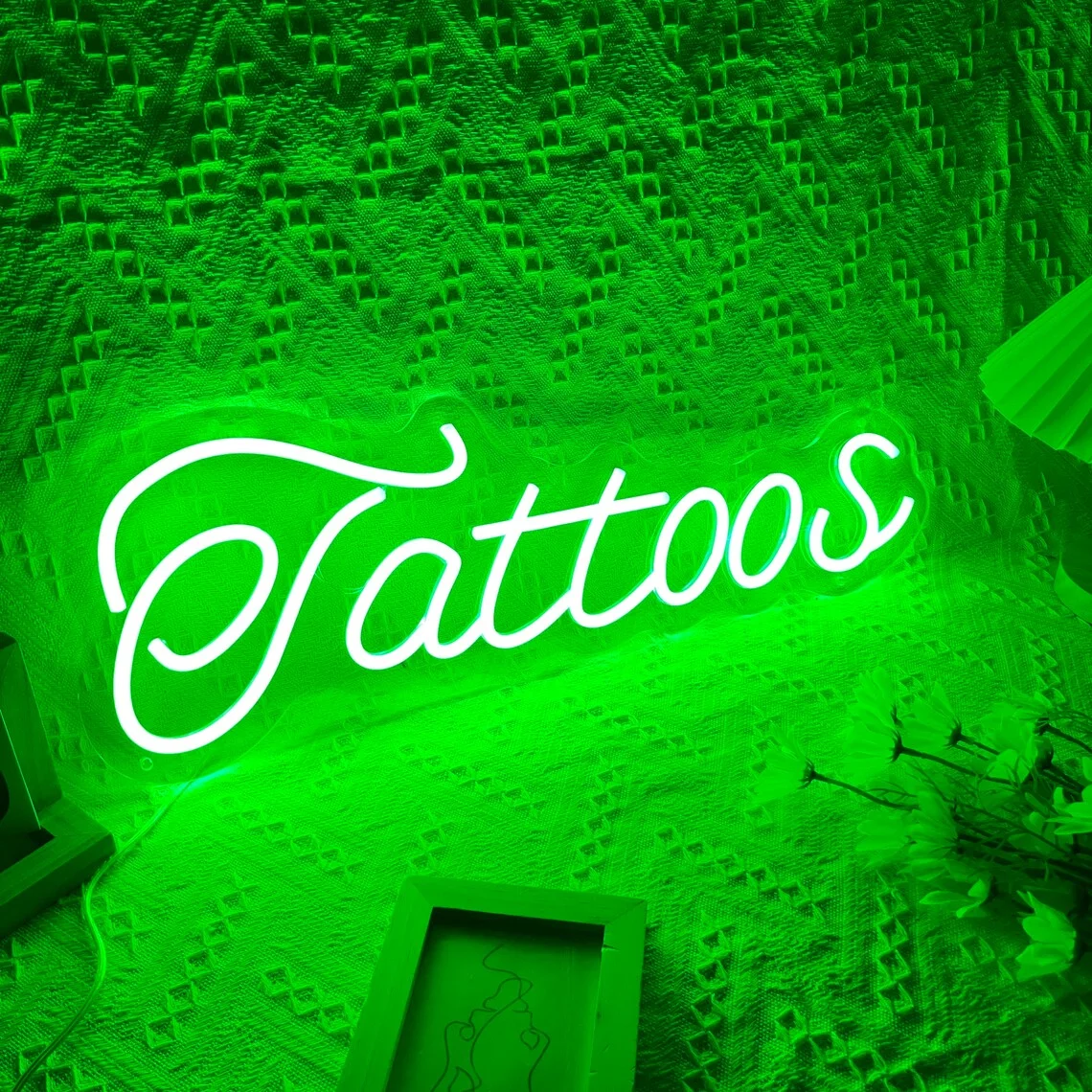This highly detailed photograph features a chair draped with a lacy, diamond-textured blanket, enveloped in a vibrant neon green glow. Centered prominently on the chair is a white-colored, neon-like sign reading "tattoos" in a cursive font, which is the only white element in the image. The sign casts a luminous green hue over the entire scene. Accompanying the sign are a variety of objects: a small tray, a bouquet of white flowers situated towards the bottom right of the chair, and a frilled lampshade just visible towards the upper right-hand side. Additionally, a wooden-framed portrait and another wooden object are seen on either side of the chair. The soft, intricate texture of the lacy blanket forms a backdrop to this eclectic arrangement, creating a compelling visual contrast against the neon-lit ambiance.